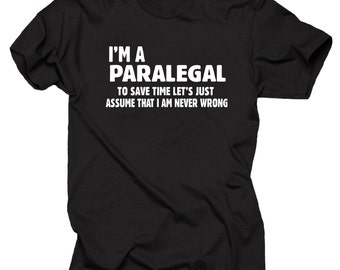This image features a black, short-sleeved t-shirt laid flat against a pure white background, emphasizing the shirt in an isolated shop-like display. The t-shirt has a humorous inscription in white sans-serif font, which stands out vividly against the black fabric. The prominent text at the chest reads, "I'm a paralegal," in a large, bold font spread across two lines and left-justified. Below this, in a smaller font size and centered, it continues with, "To save time, let's just assume that I'm never wrong." The t-shirt appears to be a casual crew neck, although the very top where the neck opening would be is cut off from the image. The short sleeves extend outwards on both sides with noticeable creases on the body, suggesting a relaxed fit, typical of a block-style t-shirt often worn by men. The detailed layout and distinctive text add a humorous touch to this otherwise standard t-shirt design.